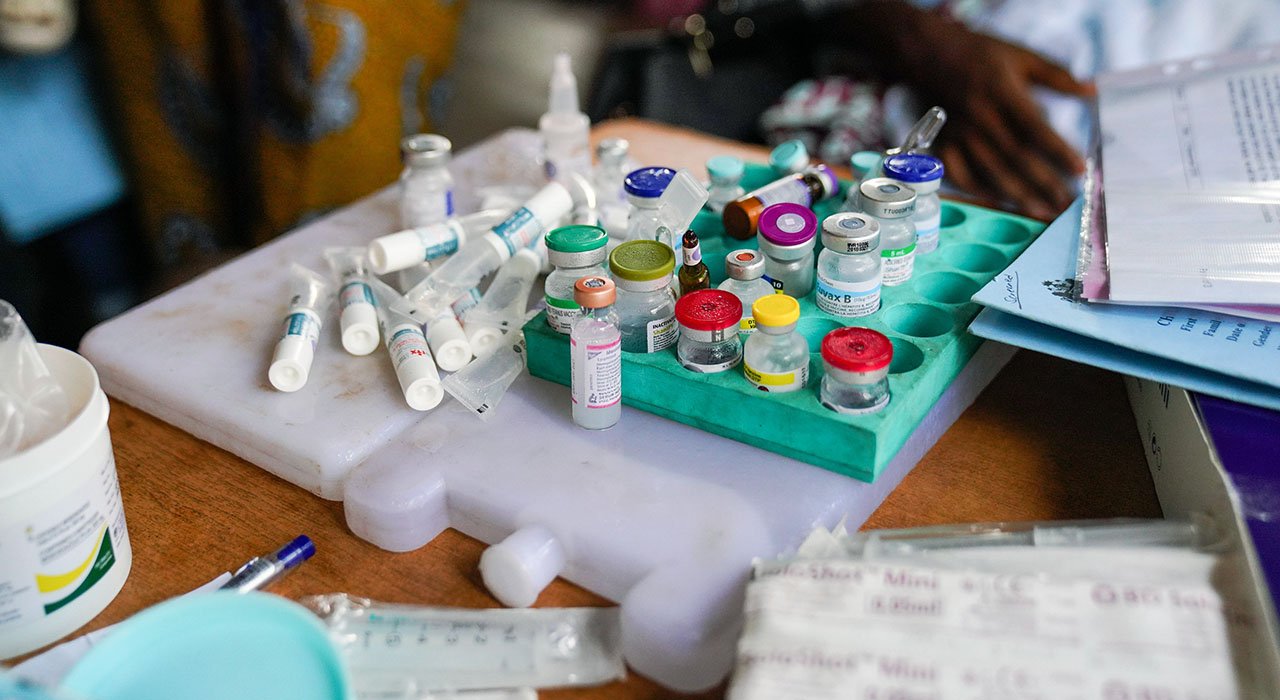This photograph captures a chaotic medical workspace, possibly in a doctor's office or phlebotomist's area, characterized by an array of disorganized medical supplies scattered across a wooden surface. Prominently featured are several small glass vials filled with clear liquid, suitable for needle injections, and small plastic tubes resembling containers you'd twist open. On the left side, there are packages of syringes and some injecting tubes, which are white and clear. A blue pen and more cylindrical plastic containers are visible towards the bottom left corner. In the front, there's a container of mini band-aids, while on the right, a stack of medical forms and papers can be seen. A hand clad in white clothing and some folders appear faintly in the background, contributing to the disordered impression of the scene.